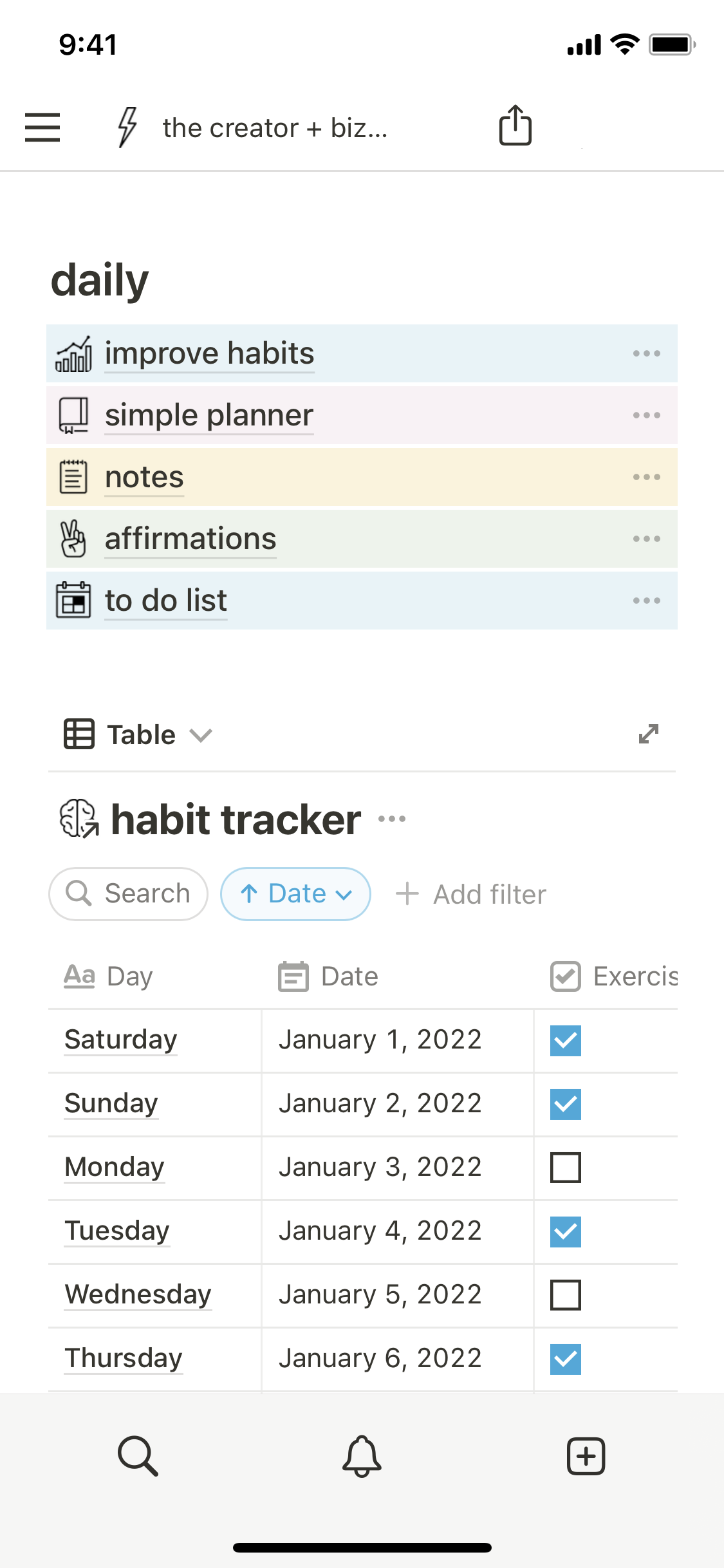A screenshot of a life-tracking app interface is displayed on a predominantly white background. The interface features a navigation bar at the top, which may double as a search bar. The main section is organized into various interactive lists and tables. The first area is labeled "Daily," offering several clickable links: "Improve Habits," "Simple Planner," "Notes," "Affirmations," and "To-Do List."

Below this section is a "Habit Tracker" table that shows each day of the week, starting from January 1st, 2022. The table includes check marks for certain days, indicating completed activities; for instance, the user exercised on all days except Monday and Wednesday.

At the bottom of the interface, three icons are visible: a magnifying glass likely for search functionality, an alarm button possibly for setting notifications, and a plus button whose function is unclear but may involve adding new tasks or goals. Overall, the app is designed to help users track their activities and improve their daily habits with potential notifications for maintaining consistency.